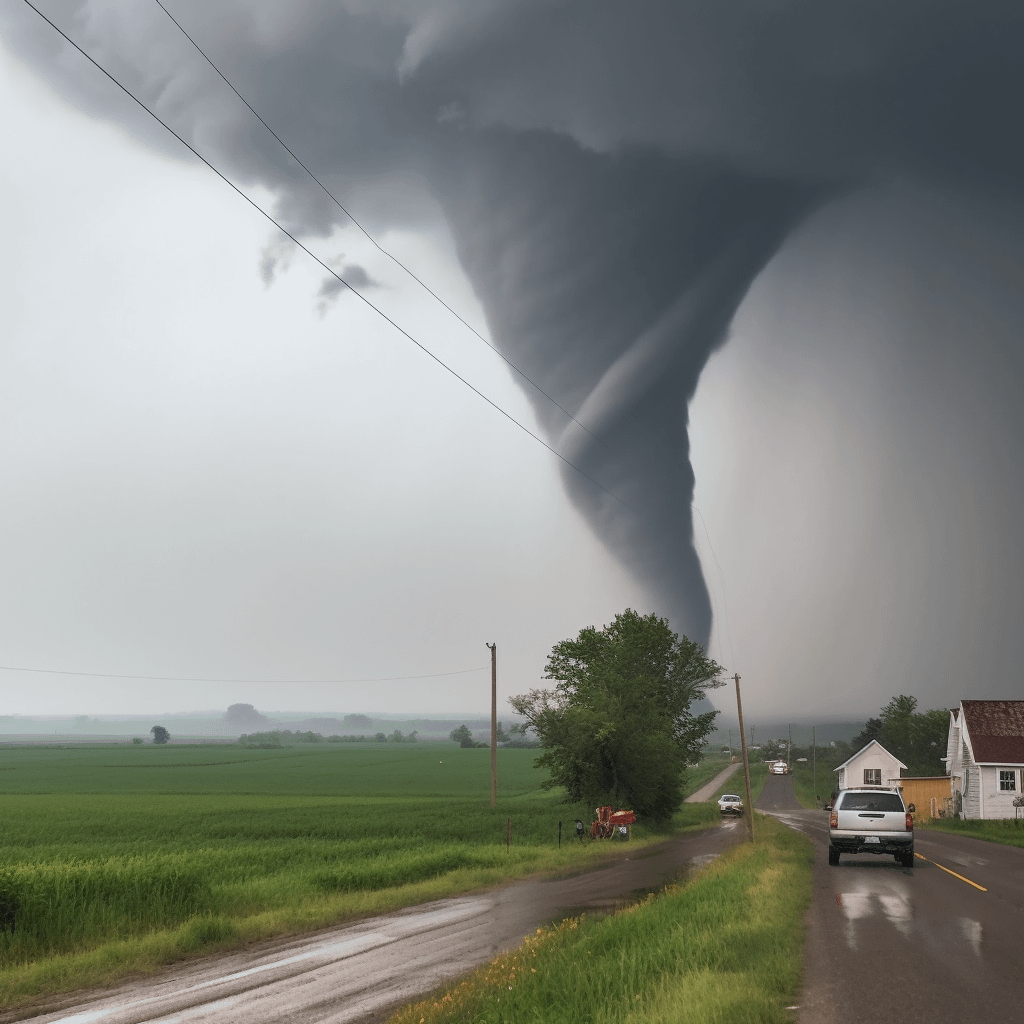This photograph captures a dramatic and intense scene of a large, perfectly formed tornado ripping through a green field. The tornado, characterized by its classic cone shape, is massive at the top, tapering into a smaller, more defined funnel at the bottom. The sky is dark and gloomy, completely overcast with no hint of blue, creating a spooky and almost apocalyptic atmosphere. Rain is falling heavily, particularly evident on the right side of the image, adding to the grim ambiance.

In the foreground, there is a wet road with a couple of cars that appear to be perilously close to the tornado’s path. Small white houses line the street to the right, while the open field stretches to the left. Overhead, power lines crisscross the sky. The right side of the image also includes a large tree and a tractor, which emphasize the normalcy of rural life disrupted by the monstrous funnel cloud. Silhouettes of more houses and objects can be seen in the background, engulfed by the gray, ominous sky. The scene suggests imminent danger to the cars and houses that lie close to the tornado’s destructive path.